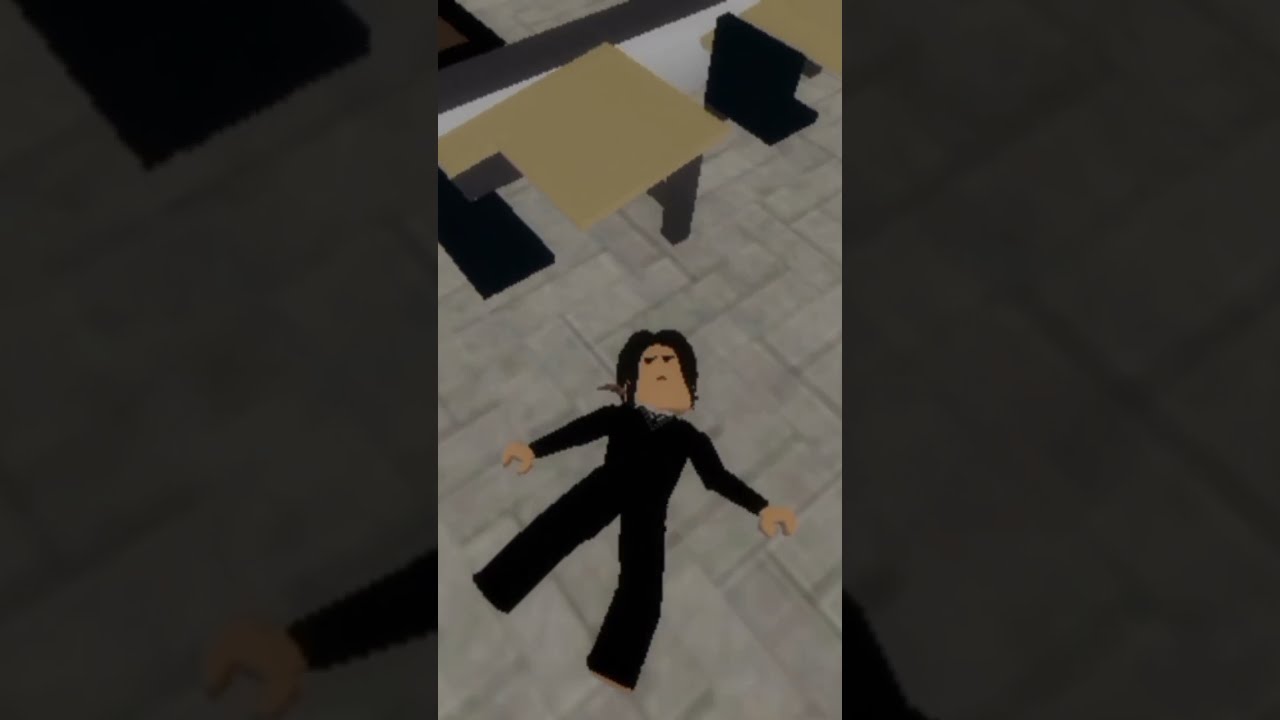The image appears to be a still frame from a video game, potentially resembling popular games like Minecraft or Roblox due to its 3D cartoonish style. The central focus is on a character lying on a partially tiled, gray concrete floor, with arms splayed out. The character has white skin, black hair, and is dressed in an all-black outfit. The floor surface displays various gray tiles and appears slightly blurry at the bottom.

In the scene, there are two upturned desks, one of which has an upside-down black chair with an orange top nearby. These elements give the surroundings a chaotic feel, suggesting an incident or a game scenario where the character may have fallen or been hit. The layout includes side borders that replicate and magnify the central image but with a shadowy overlay. The image's vertical orientation and framing indicate it was captured on a phone, with the primary subject sharply focused in the center, while the left and right sides remain blurred, giving a zoomed-in effect.